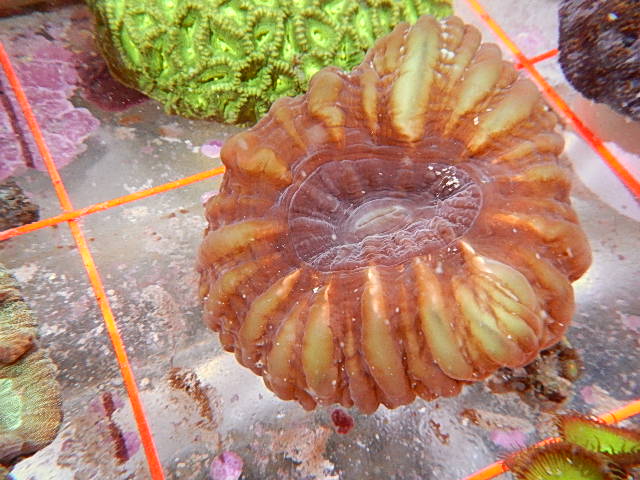The photograph presents a close-up of a collection of different rocks, with a focus on a brown rock and a partially visible green, rough-textured rock next to it, positioned on an opaque glass surface accented with orange trimming. While the scene does not include identifiable features such as dates or people, the setup suggests a display, possibly within an aquarium or a specialized showcase, given the presence of orange roping that seems to segregate each item. The detailed elements include the noticeable colors and textures of the rocks – particularly brown, green, yellow, and orange hues – which hint at a studied, almost curated arrangement.